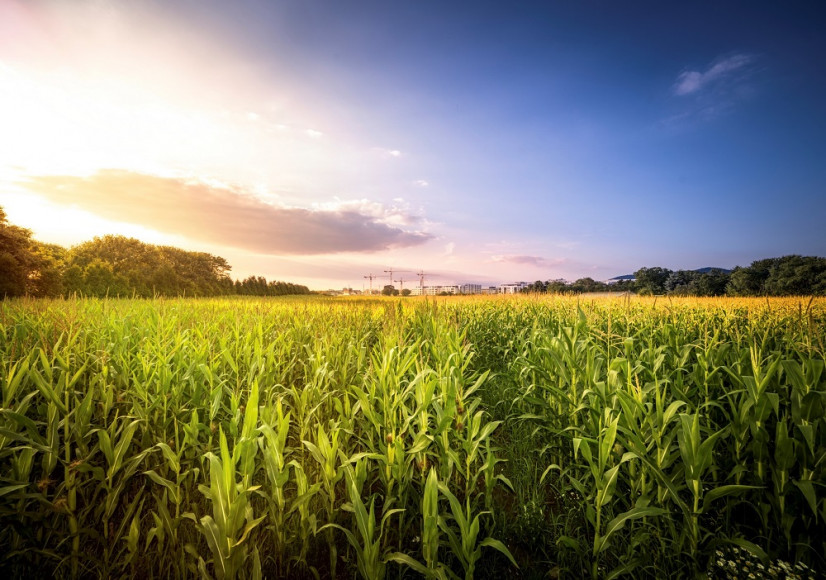This is a vibrant, colored photograph, possibly an AI-generated image, depicting a vast cornfield that stretches endlessly across the landscape. The foreground features rows upon rows of young, green corn plants, which transition to a beautiful golden hue as they extend toward the horizon. The sky above displays a stunning gradient, with the left side illuminated by a bright, yellowish-white sunrise or sunset, and the right side deepening into a dark navy blue with hints of pale blue and orange in between. High in the distant horizon, a forest flanks both the left and right sides, framing faintly visible buildings in the center that may be part of a farm. These buildings are complemented by three tall towers or construction cranes that stand prominently above the other structures. The entire scene is rich in contrast and color, creating a picturesque and serene depiction of a quintessential Midwestern agricultural landscape.